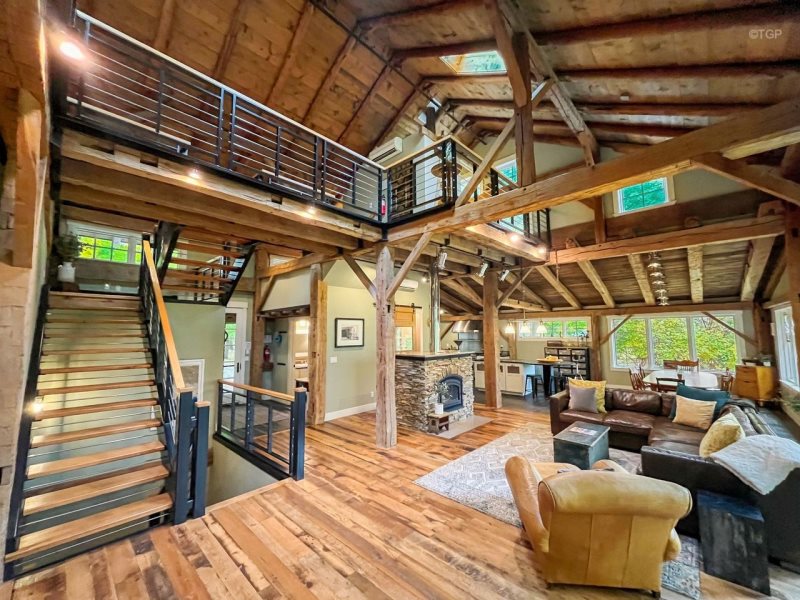The interior of the house features a rustic and modern open-plan design, emphasizing natural wood elements and industrial accents. The high ceilings are supported by exposed wooden beams, contributing to a cabin-like feel, while large, bare windows flood the space with light and offer views of lush green trees outside. The main level showcases a diverse hardwood floor adorned with a rug and furnished with a spacious brown leather sectional and a smaller yellowish leather armchair nearby. A stone fireplace, subtly hinting at brickwork, stands at the center of the room, dividing the living space from a compact kitchen area behind it. To the left, wooden stairs with black railings lead to an upper level with balconies, further enhancing the open layout. This meticulously clean and new-looking space manages to blend rustic wood elements with industrial design seamlessly, even incorporating a skylight that adds to its airy and inviting atmosphere. The overall scene gives an impression of a meticulously designed and possibly computer-generated image due to its polished appearance.